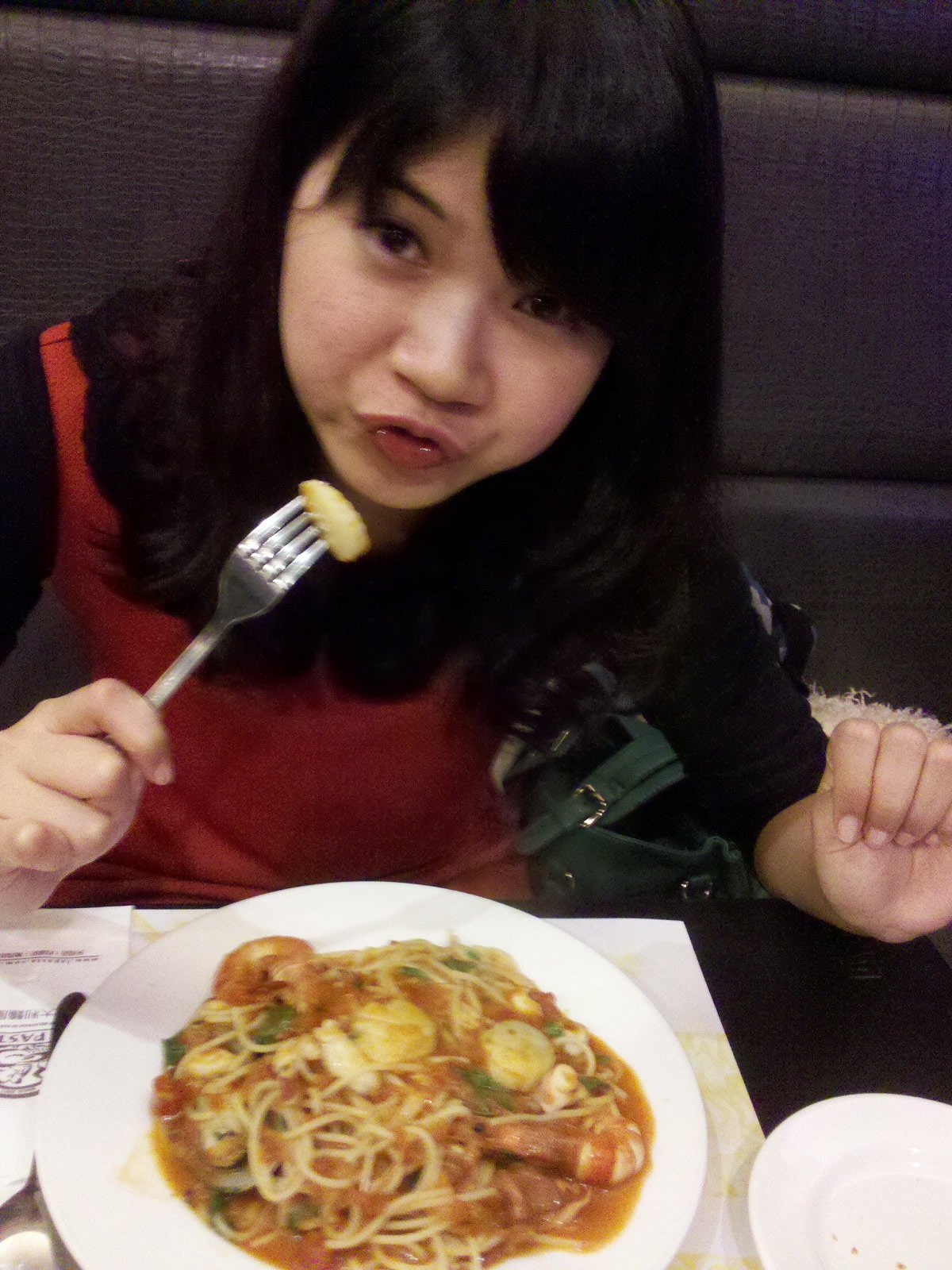In the vertical, rectangular image, a young Asian woman with straight, dark brownish-black hair cascading over her eyebrows and shoulders is captured mid-meal. She is seated in a dark gray cushioned booth at a dark brown table. Dressed in a red and black ensemble— a black top with a red tank top over it, featuring black sleeves that extend to her elbows—she playfully tilts her head and makes a duck lips face. A dark green bag rests beside her on the booth.

In front of her, a white plate holds a dish of pasta mixed with various seafood, possibly shrimp and scallops, along with green garnishes, all covered in a red sauce. She holds a fork with a piece of food close to her mouth, preparing to take a bite. Next to the main plate, there is a smaller white plate and another utensil peeking out from underneath. A piece of paper, likely a receipt, is also visible near her plate. The image captures a casual, lighthearted moment as she enjoys her meal.